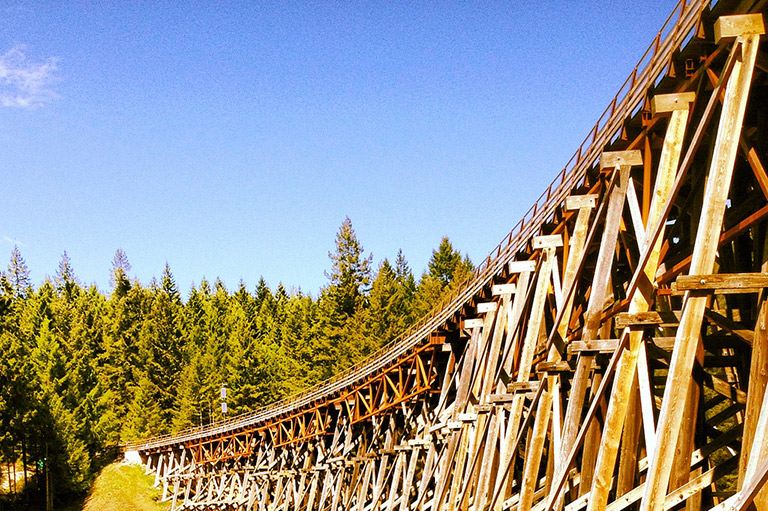This outdoor image captures a stunning perspective from the ground looking up, showcasing a majestic wooden train trestle that dominates the foreground. The trestle spans from the top right corner of the image, diagonally down to the lower left. Its intricate structure is comprised of numerous support beams and crossbars, all crafted from a dark brown, copper-toned wood. The top of the track is subtly hinted at, with parts of the railing visible but not the track's surface.

The backdrop is a vibrant blue sky, punctuated in the top left corner by a small, wispy white cloud. Below, a dense expanse of very tall, green pine trees stretches across the image. While some of the tree trunks are visible, the focus is primarily on the individual peaks of the towering pines, with five trees distinctly taller than the rest. These trees vary in height, creating a visually dynamic forest that blends seamlessly together. The image captures the serene beauty of nature interwoven with the rustic charm of the wooden trestle, inviting viewers to admire the harmony between man-made and natural elements.